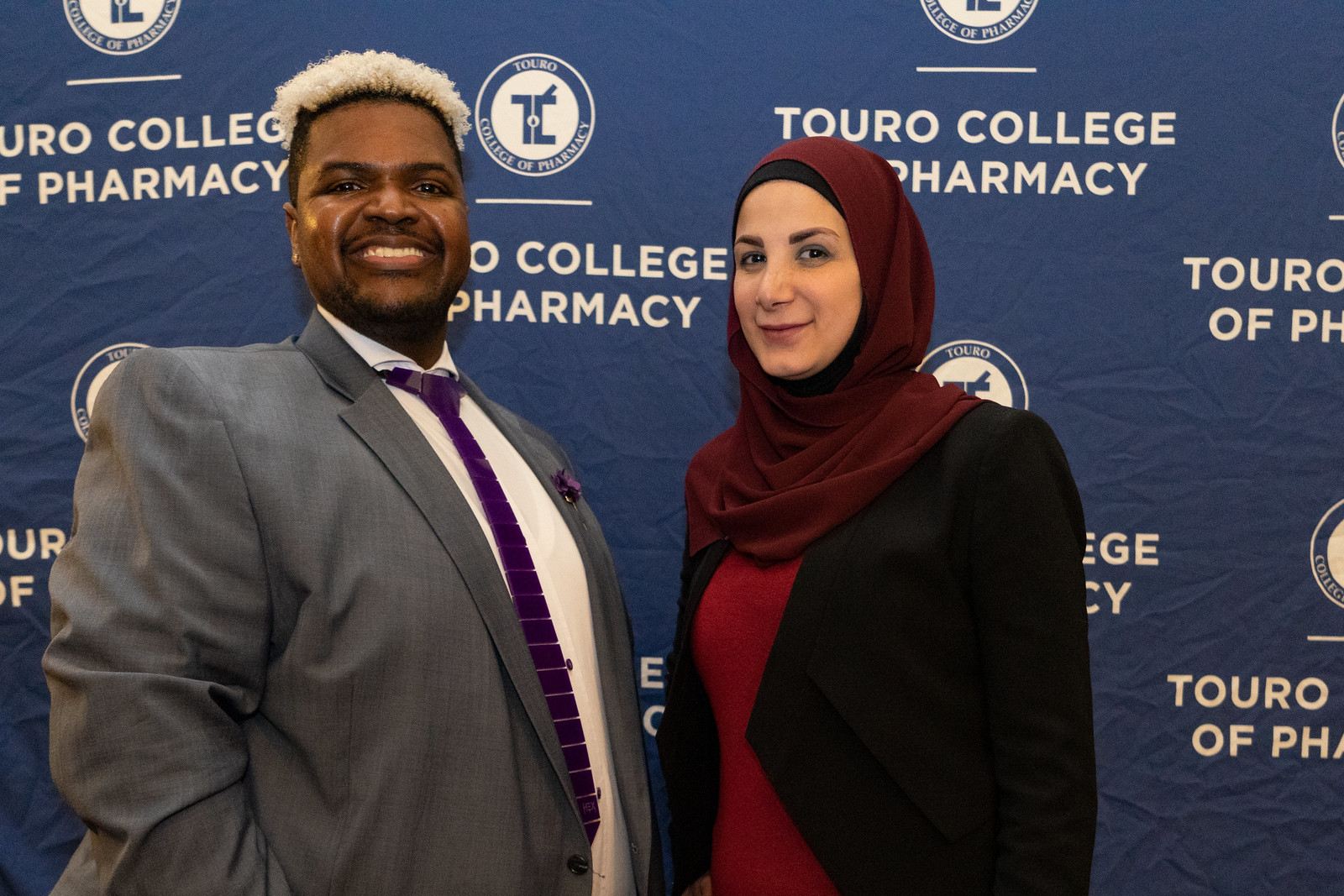This image features two individuals smiling and posing in front of a blue fabric sign that bears white text reading "Touro College of Pharmacy," with the emblem of the college, resembling a T shaped like a pharmacy symbol, prominently displayed above it. The man on the left is a tall black gentleman with dyed blonde hair, wearing a gray sports jacket, a white undershirt, and a distinctive purple tie adorned with noticeable lines. The woman on the right, who appears to be of Middle Eastern descent, is donned in a red hijab and red sweater, complemented by a black jacket. The blue background is somewhat creased and repetitively features the Touro College of Pharmacy logo, consisting of a small white circle with a bold blue border and symbols resembling back-to-back letter Cs with a line emerging from one of them.